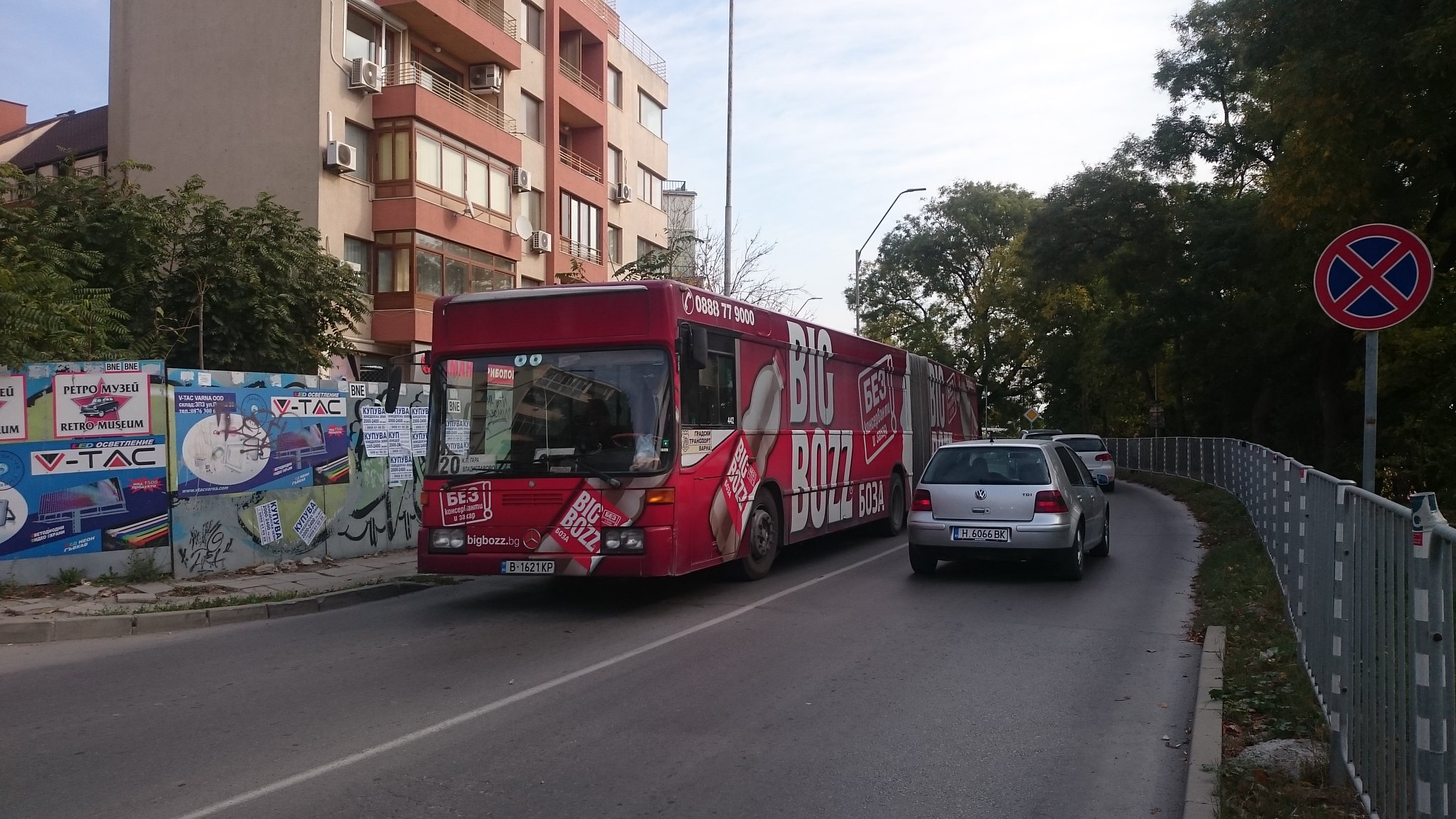This is a color photograph capturing an urban street scene with a prominent red bus heading towards the left side of the image. The bus, a double articulated type with a spring-like structure in the middle, features multiple advertisements. It has white lettering and an image of a bottle with brown liquid inside, a red cap, and the label reads "Big Boss Goza" and "Big Buzz 6038." The front of the bus displays the number "0888779000" in the top corner, a "20" on the windscreen, and a Mercedes logo with "BigBoss.BG" beside it. The bus's number plate reads "B162KP."

Opposite the bus, on the other side of the wide grey road with a central white line, is a silver Volkswagen car driving to the right, bearing the number plate "H6066BK." Another vehicle is visible beyond it. To the right edge of the road, there is a narrow curb leading into a strip of grass, beyond which stands a metal fence. On the fence, a tall pole holds a traffic sign: a red circle with a red X forming four inward-facing triangles in dark blue.

In the background, there’s a dark green forested area of trees. The left side of the image features a block of beige apartments with terracotta-colored balconies. The wall below the balconies is adorned with colorful photos or stickers in blue and green, with partially visible text including "TAC" and "Retro Museum." Additional foliage and trees are present in front of the apartments. Street lights line the road, and the sky transitions from blue to white in the middle, with some wispy clouds scattered across.